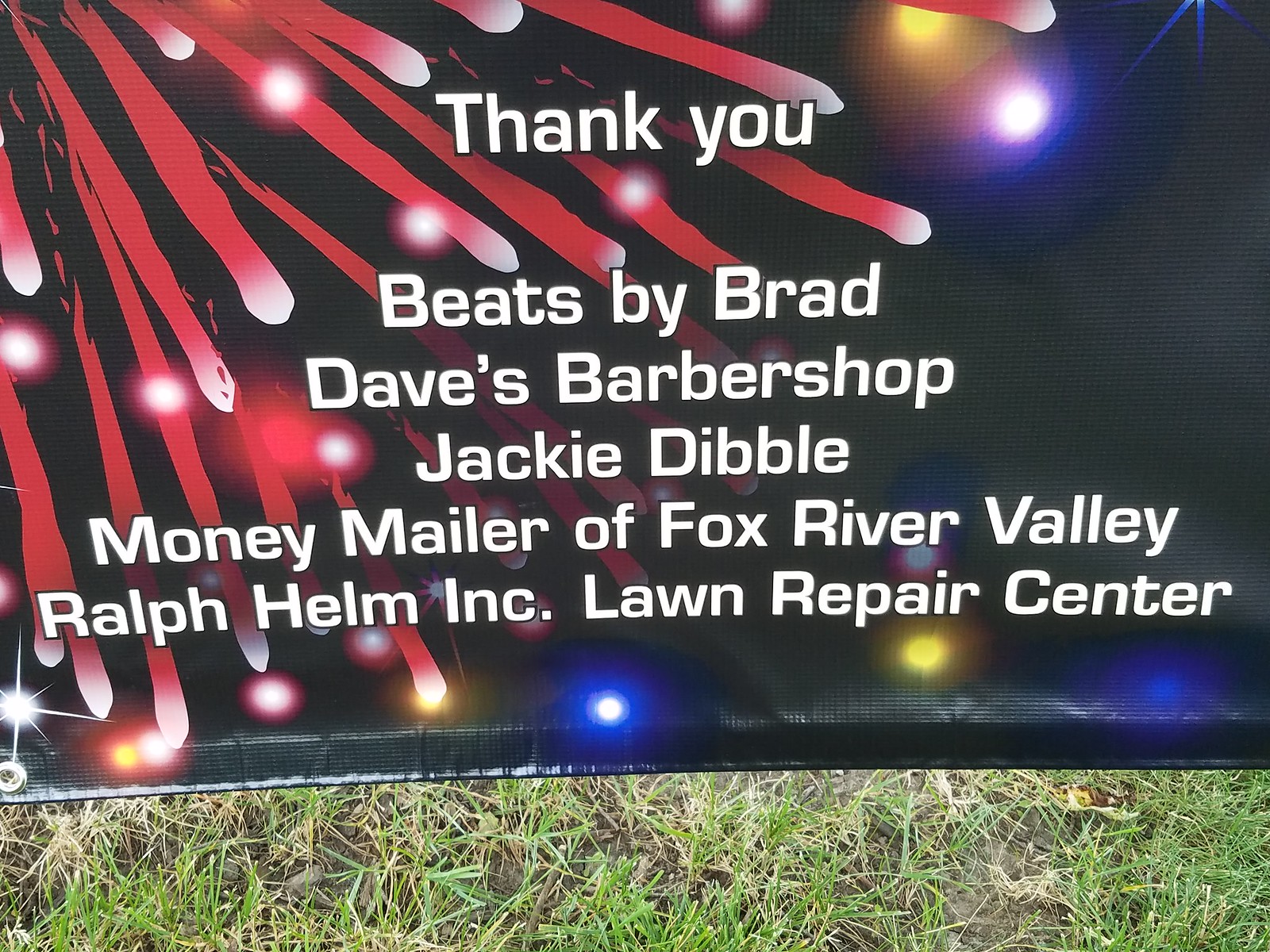The image features a prominent banner with a black background, adorned with an array of colorful lights in hues of blue, green, pink, yellow, and red. Streams of red streaks with white-tipped ends, resembling fireworks or rocket trails, are seen shooting downward, particularly from the top left corner. Below the banner, a grassy area with visible patches of brown dirt is noticeable, indicating less-than-healthy grass. The banner displays a heartfelt message in bold white letters that reads: "Thank you Beats by Brad, Dave's Barbershop, Jackie Dibble, Money Mailer of Fox River Valley, and Ralph Helm Inc. Lawn Repair Center." A faint, shiny light with three radiating lines is situated in the top right corner, adding an extra sparkle to the scene.